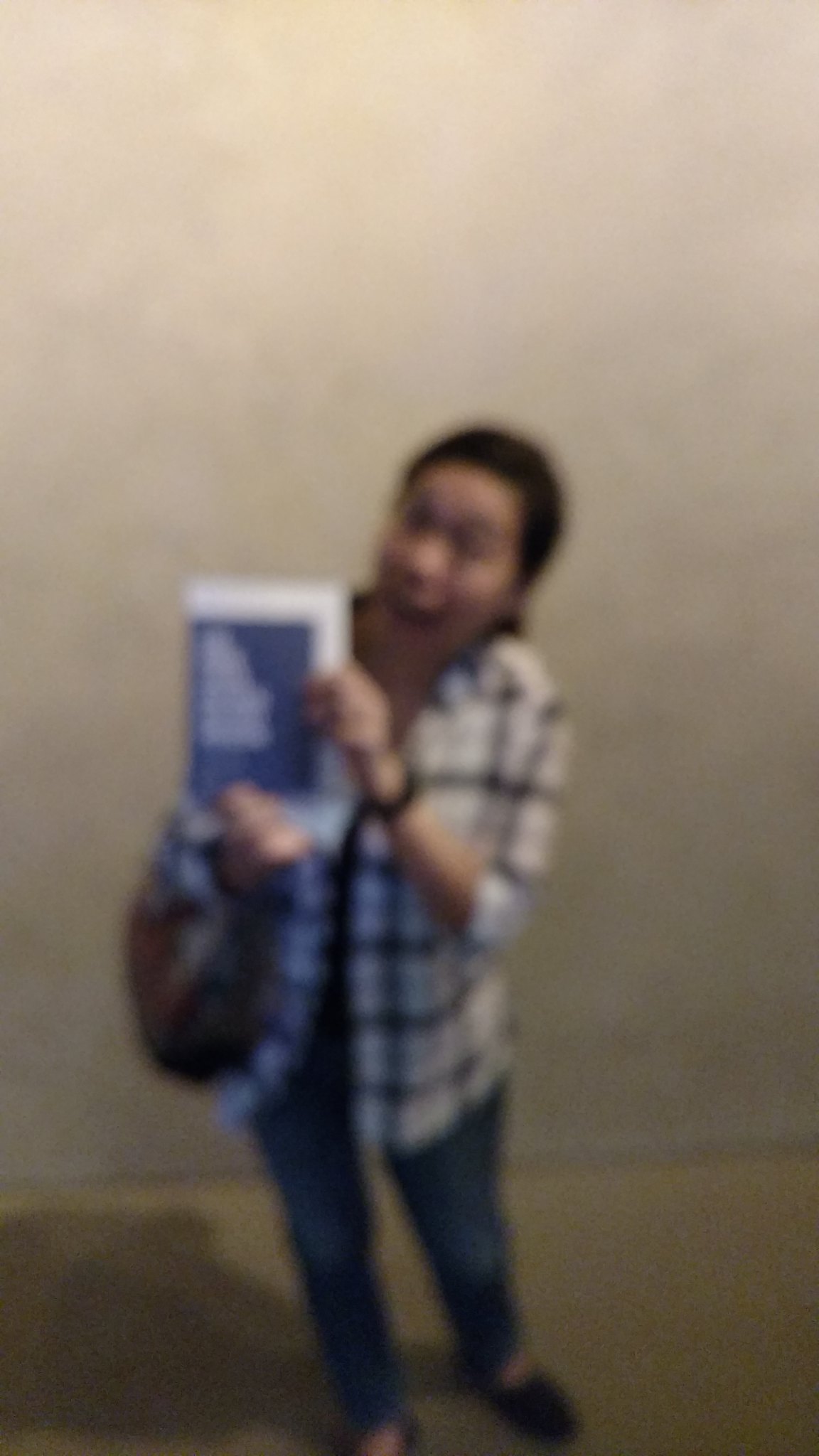In the image, a woman is positioned in what appears to be a beige-brown room. The photo is quite blurry, yet certain details are discernible. The woman’s face exudes excitement, characterized by what seems to be an open-mouth expression. She has dark hair that is pulled back, and she appears to be of Asian descent. She is dressed in a light-colored or white plaid shirt with buttons, which are undone, revealing a dark-colored shirt underneath. She also wears blue jeans that fit her mid-range, neither overly loose nor too tight, along with black shoes. On her left arm, she carries a large purse or bag, and she holds a blue book or pamphlet with a white border and some white text off-center to her left.